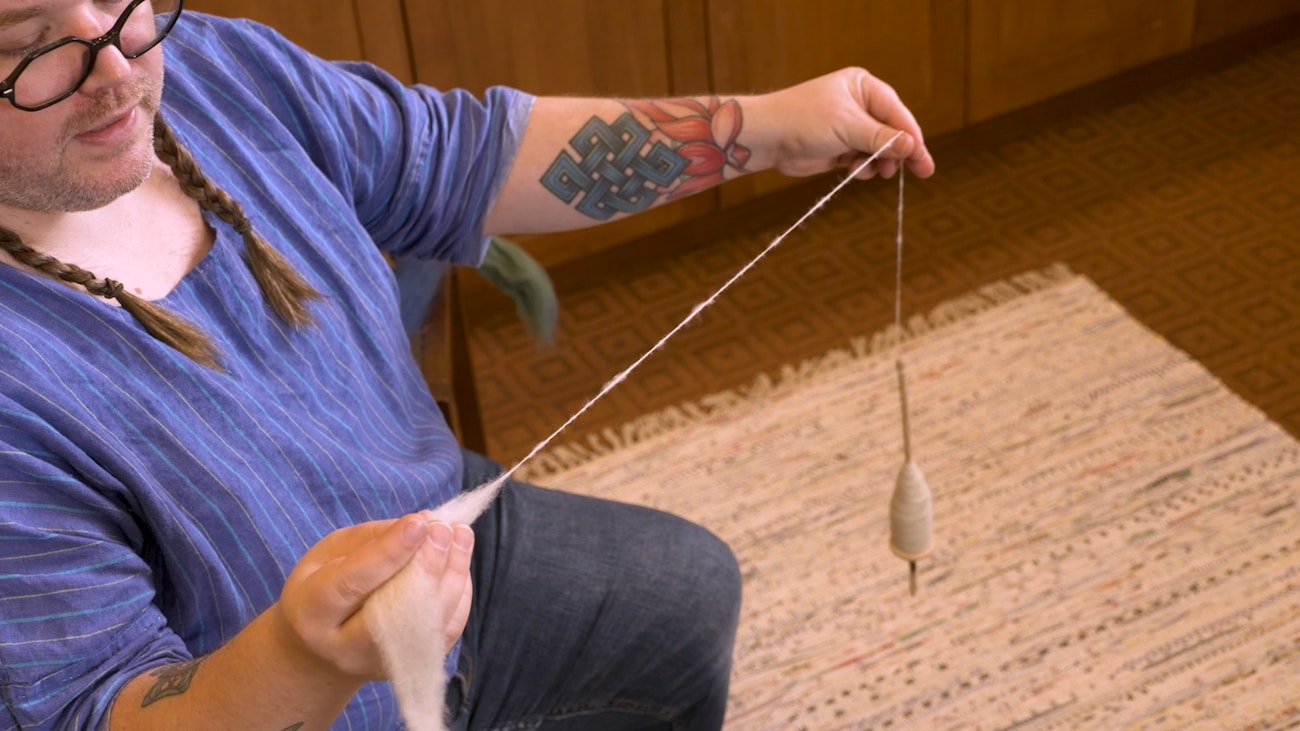In the photograph, a man with braided pigtails is diligently spinning wool into yarn without the aid of a spinning wheel. He uses a spindle resembling a dreidel, which hangs from fibers attached to it. In his right hand, he holds a shock of white wool, and the twisted wool threads move toward his left hand, which is spinning the spindle. He is dressed in a blue top and gray or black pants, with black-rimmed round glasses perched on his face, and a five o'clock shadow covering his beard and mustache. His left forearm displays a dark green Celtic-style cross tattoo, with an indistinct red tattoo situated between the cross and his wrist. The setting appears to be indoors with a dark brown floor partially covered by a white rug with tan fringes. The background features wood paneling or cabinetry, adding a warm, rustic feel to the scene.